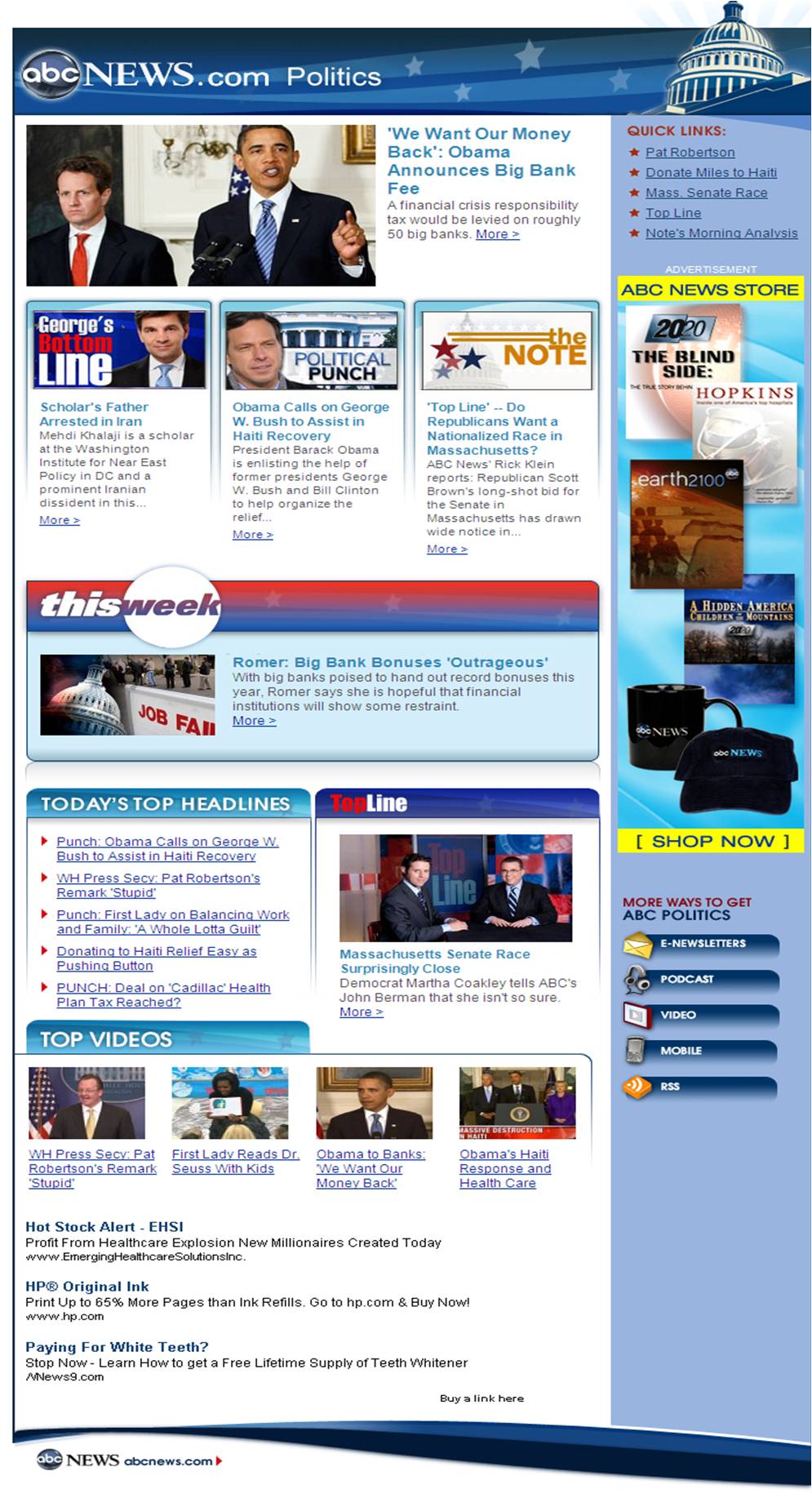An image depicts a blurry news webpage from abcnews.com under the politics section. In the image's focal point, former President Barack Obama stands beside a caucasian man dressed in a black suit, white shirt, and red tie. The headline beneath the picture reads, "We want our money back, Obama announces big bank fee." Subtext includes partial and unclear phrases such as "George something line, political punch," and "this week," followed by various indistinct text. The page also highlights "Today's Top Headline" with additional blurred text below it. Further down, the "Top Videos" section features four thumbnails, each accompanied by illegible descriptions. On the right side of the page, a segment labeled "ABC News Store" includes a "Shop Now" button and more unreadable text.